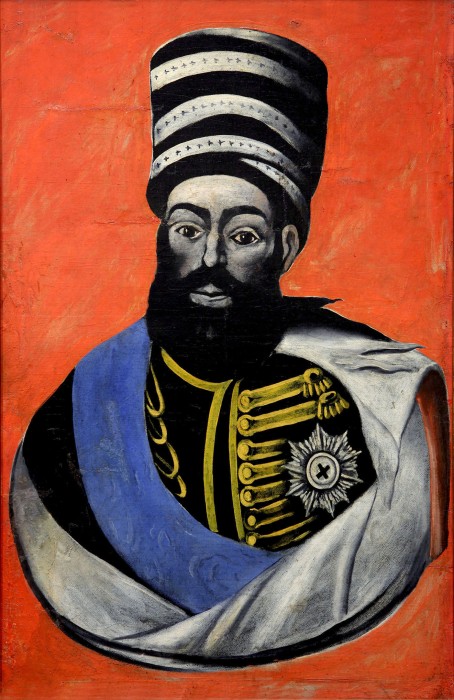In the center of this vertically oriented image is a detailed drawing or painting of a man, possibly a ruler, king, or czar. The background is predominantly red with visible smears of light gray and orange brush strokes, giving it a textured, painted appearance. The man has a thick black beard and mustache, black eyebrows, and high cheekbones. He wears a tall black hat adorned with three horizontal silver strips.

His attire includes a black military-looking jacket with gold buttons and a gold design, featuring gold epaulets on his shoulders. Draped over his outfit is a blue and black sash on the left side, and grey cape-like material on the right. Additionally, a silver star embellishment resembling a badge is displayed on the front of his uniform. The man gazes directly ahead with a neutral expression, all elements combining to suggest his regal or authoritative status.